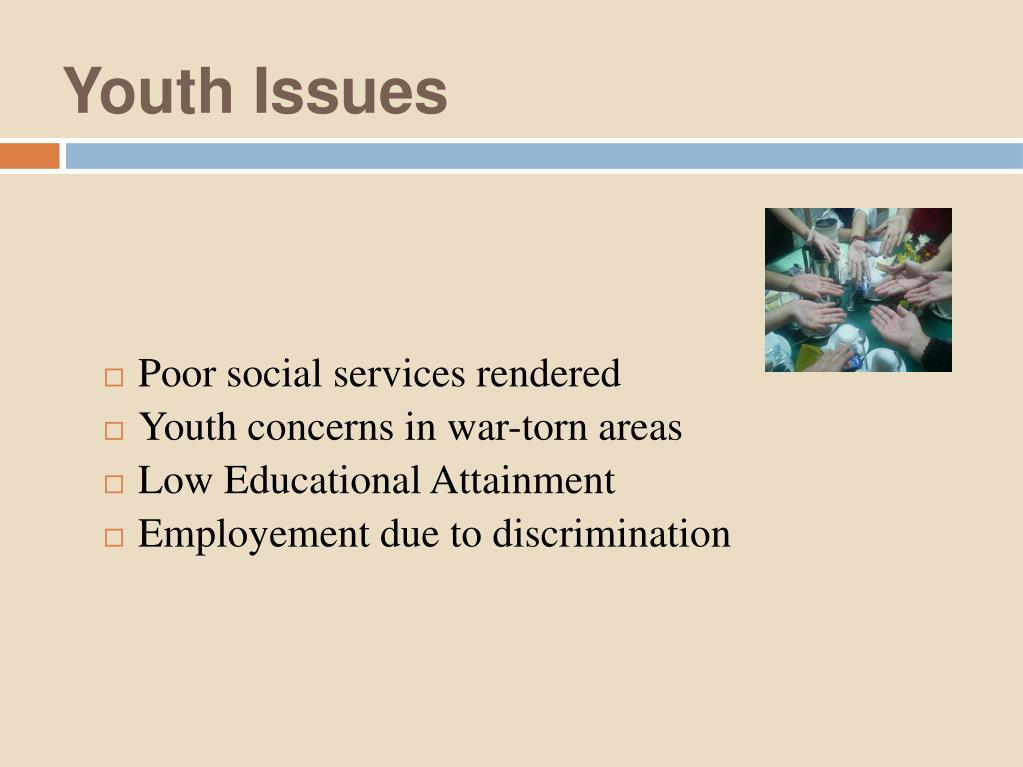The image, resembling a PowerPoint slide with a light beige/tan background, prominently displays "Youth Issues" in brown lettering at the top left. Underneath this heading is a horizontal bar extending across the slide, transitioning from orange with a white border on the left to light blue with a white border on the right. To the right of the bar is a small square photograph featuring around ten white hands arranged in a circle, all with their right palms facing upwards into the center. Below this photograph, four bullet points are listed in black text with empty orange square indicators on the left. The points read: Poor Social Services Rendered, Youth Concerns in War-Torn Areas, Low Educational Attainment, and Employment Due to Discrimination.